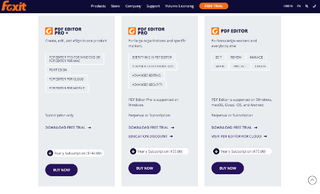The image presents a pricing comparison for a service called "Pro Editor," featuring three distinct columns: "Pro Editor," "Pro," and "Pro Editor (again)." Each column outlines different tiers of the service with varied features. The layout is displayed on a light blue background, although the text is somewhat blurry, making it challenging to discern finer details. Key elements include an orange "G" icon and the word "FOXIT" in the top left-hand corner, possibly indicating the brand or platform. Additional details are presented in an orange box within the image. At the bottom of the image, there is an option to "Pay Now" for the selected service tier. The comparison seems to suggest that the "Pro Editor" offers the most comprehensive set of features and the best value for money compared to the other options.